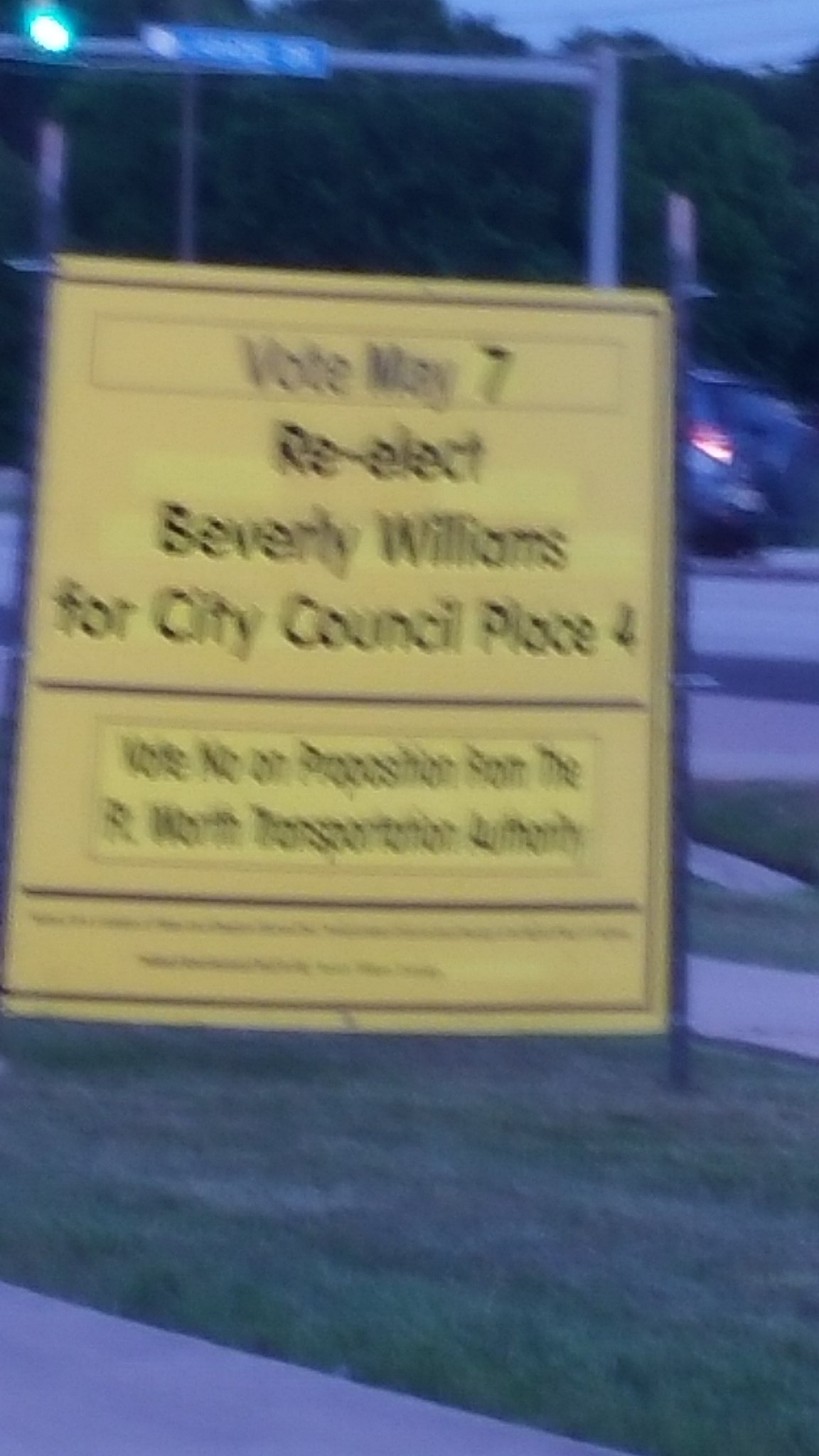In the midst of a bustling street or a spacious car park stands an eye-catching hoarding, or large notice, prominently conveying a political campaign message. The sign, an attention-grabbing yellow, is mounted securely on a sturdy frame. It boldly states "Vote May 7, Re-elect Beverly Williams for City Council Place 4" in striking black lettering. Below this primary message, a smaller boxed section also contains text in black on the yellow backdrop, though the details are blurred and difficult to decipher. Despite the unclear smaller print, the main message remains clear, marking this notice as a significant promotional material for Beverly Williams's re-election campaign.